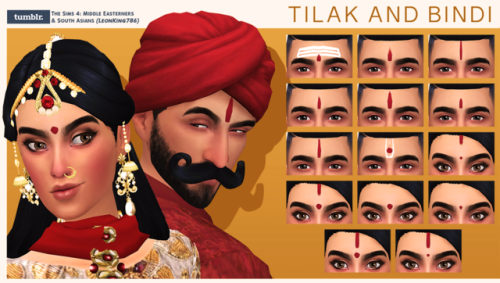The image is a banner graphic from Tumblr featuring The Sims 4 Middle Easterners and South Asians customization options. At the top, a beige bar spans across, displaying the Tumblr logo on the left and reading "The Sims 4 Middle Easterners and South Asians" in small, dark text beside it. In striking gold text on the right, it says "Tilak and Bindi." The left side of the banner showcases two 3D avatar illustrations resembling Sims characters. The female avatar has fair skin with pinkish cheeks, black eyebrows, and eyes, adorned with a gold nose ring, a red bindi between her eyebrows, and black hair. She wears traditional Middle Eastern or Indian jewelry and clothing. Next to her, the male avatar sports a red turban, dark brown eyebrows, a thick handlebar mustache, a thick beard, and a vertical red tilak on his forehead. On the right side of the banner, a grid displays 18 different thumbnails demonstrating various bindi and tilak designs on foreheads. The display area for these examples has a light gold-colored background and is clearly labeled "Tilak and Bindi." This detailed customization screen highlights the cultural attire and forehead markings options available within the game.